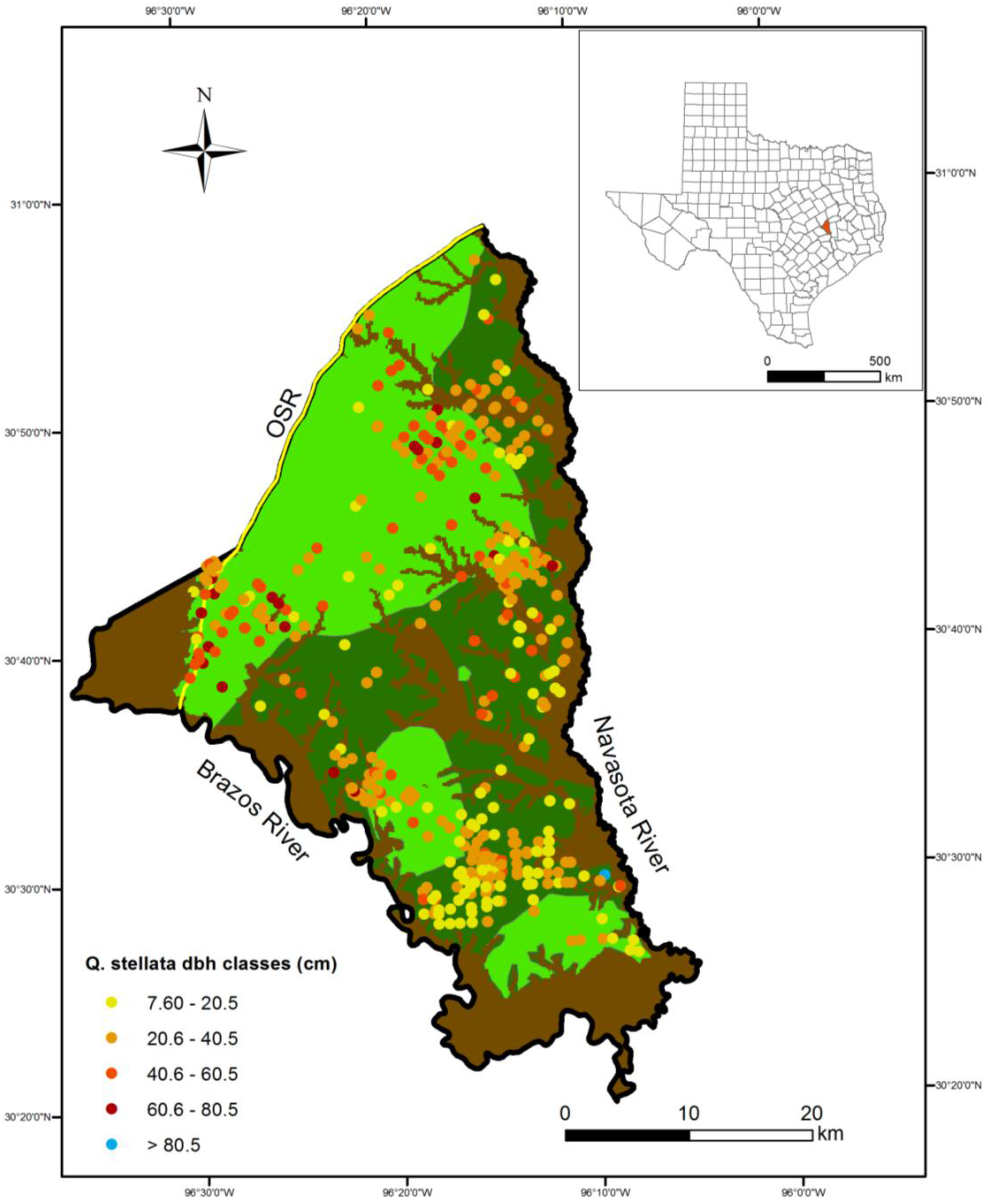This detailed image depicts a section of a map focusing on a specific region within Texas, highlighting a smaller county bordered by the Navasota River to the right and the Brazos River to the left. The map, which resembles a coordinate grid, ranges from 96°30' W to 96°00' W horizontally at the top and spans vertically from 3100 N to 3020 N. The county is segmented into various parts, with one distinct section marked in red, suggesting a focal area for study or emphasis.

The map includes a variety of colored dots indicating different classes, labeled as Stelata DBH classes. These dots come in multiple colors—yellow, orange, red, wine, and blue—each representing different data points or classifications. The map also features diverse renderings of the county's landscape, displaying brown, green, and dark green areas, further detailing the geographic and possibly ecological variances within the county. Despite the abundance of detail, the map appears to lack an explicit title or name, focusing instead solely on the cartographic representation of this Texan county and its classes.